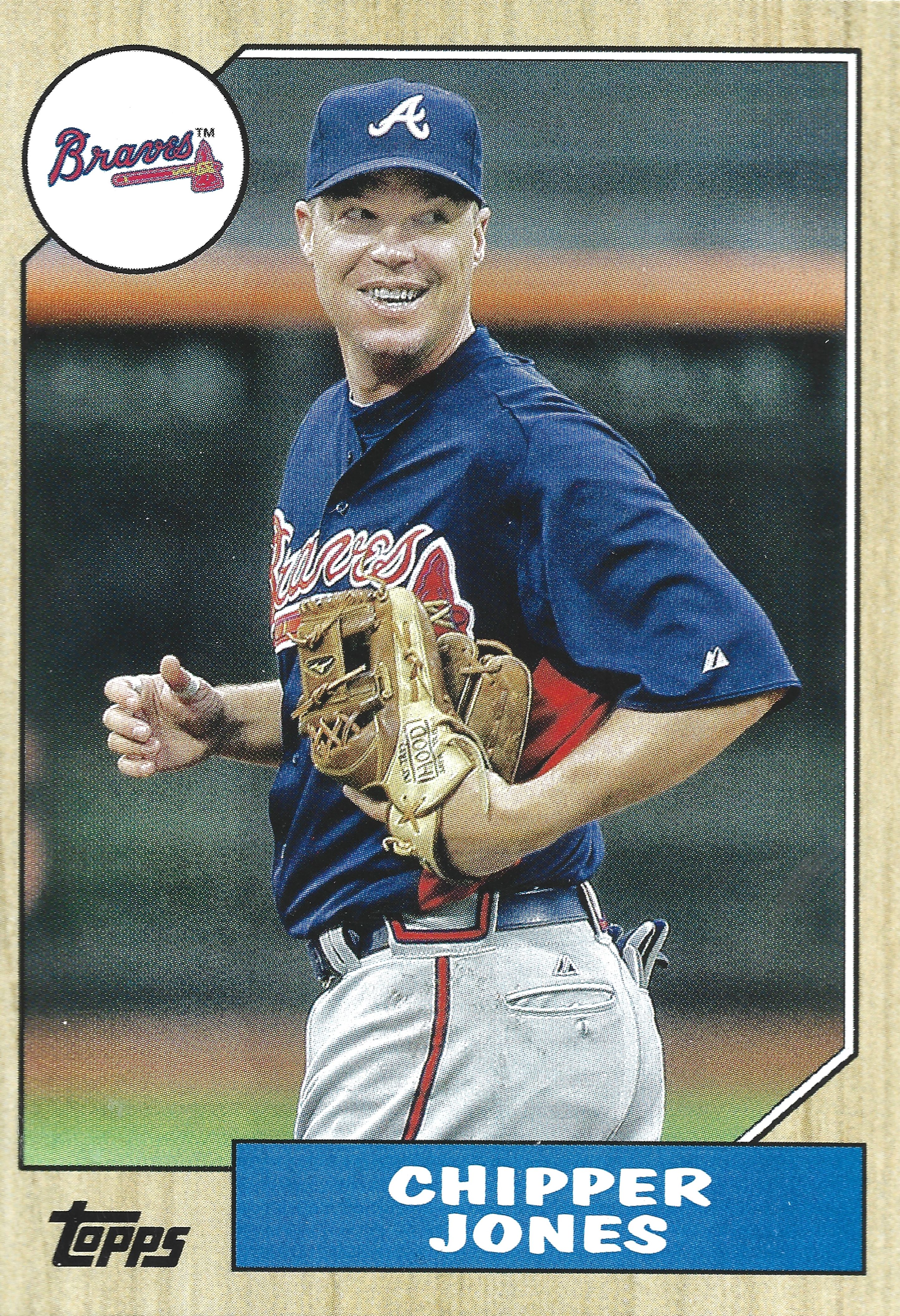This is an image of a collector's baseball card featuring Chipper Jones in an Atlanta Braves uniform. The card has a grainy printed photograph of Jones standing on the baseball field, possibly during a game. He is shown from the side, looking back and smiling. He is wearing a dark blue baseball cap with a white "A" and a matching dark blue jersey with the word "Braves" on the front. He is also wearing light gray baseball slacks with a red stripe down the side. Chipper is holding a brown baseball glove, marked with the word "Hood," up to his chest, while another glove is tucked into his back pocket. 

The card itself has a tan wood grain border with a white circle in the upper left corner that contains the Braves logo in red and blue. In the bottom left corner, there is a black "Tops" logo, indicating the card brand. His name, "Chipper Jones," is written in white on a blue rectangle at the bottom of the card. The background of the photograph features what appears to be the outfield wall, outfield dirt, and grass, adding to the authentic baseball field setting.